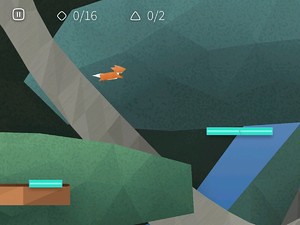The image is a screenshot from a mobile phone game featuring a level interface. Dominating the scene, a bright orange, geometrically stylized fox with a white belly, neck, and tail is leaping to the right in the center foreground. The background consists of abstract geometric shapes, primarily in shades of green and darker mossy green, which resemble large trees, and a horizontal brown wide line symbolizing a large branch or road running from the top left to the bottom right. A blue line runs from the bottom right to halfway up the screen, representing a river. In the user interface, a small white square at the top left corner contains two dashes resembling a pause symbol. To its right, a white diamond shape is followed by the text "0/16." Further right, a white triangle shape indicates "0/2." The aesthetic is highly abstract and emphasizes a polygonal art style, giving the impression that the player is either controlling or interacting with the fox in a natural, albeit stylized and abstract environment.